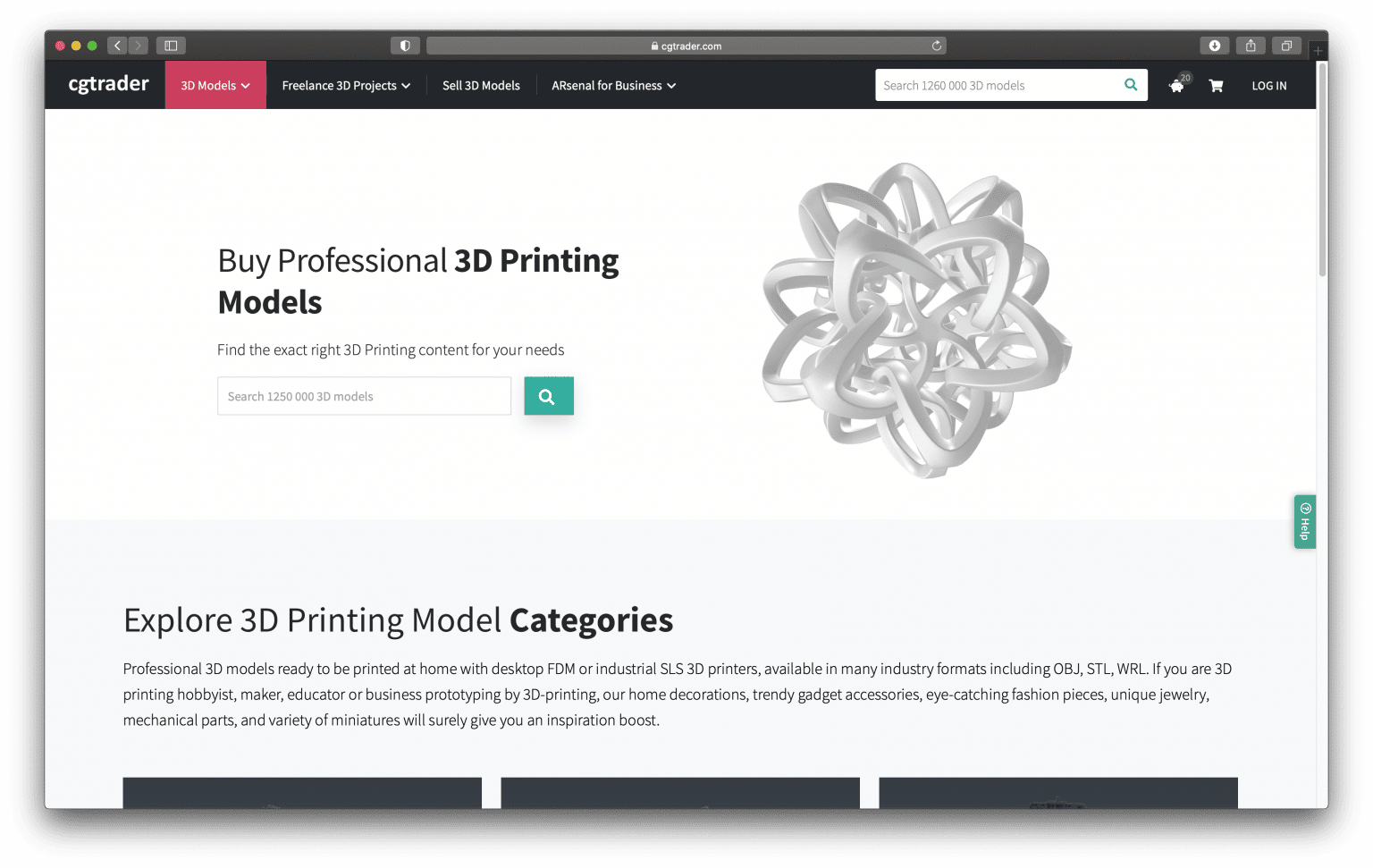The screenshot displays a computer screen focused on the CGTrader website. In the top left corner of the browser window, there are three colored buttons: red, yellow, and green, which are used to control the window. Adjacent to these buttons are the back and forward navigation arrows, followed by the address bar situated at the center. On the right side of the address bar, there are icons for download, share, and an unidentified button.

Below the address bar, the navigation menu of the CGTrader website is visible. From left to right, the menu includes several options: "Home," "CGTrader," "3D Models" (highlighted in a pinkish-red color and featuring a dropdown menu), "Freelance 3D Projects" (also with a dropdown), "Sell 3D Models," and "Arsenal for Business" (with a dropdown). To the right of these options, there is a search bar, a shopping cart icon, and a login button.

The main body of the website, set against a white background, features a prominent headline: "Buy Professional 3D Printing Models." Underneath, a subheading invites users to "Find the exact right 3D printing content for your needs," accompanied by a search bar on the right side. An image example of a 3D printed object, resembling a star or snowflake, is displayed below this text.

Further down, the text reads: "Explore 3D Printing Model Categories. Professional 3D Models Ready to be Printed at Home with Desktop, FDM, or Industrial SLS 3D Printers. Available in Many Industry Formats, including OBJ, STL, WRL." The description continues by addressing various users: "If you are a 3D Printing Hobbyist, Maker, Educator, or Business, prototyping by 3D Printing or Home Decorations, Trendy Gadget Accessories, Eye-Catching Fashion Pieces, Unique Jewelry, Mechanical Parts, and a variety of Miniatures will surely give you an inspiration boost."